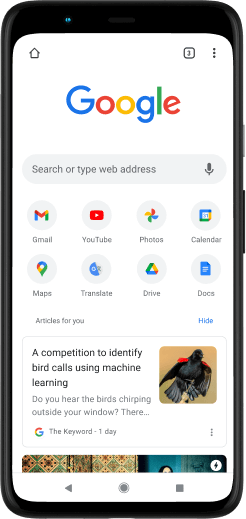A high-resolution image captures a sleek, black smartphone displaying a Google search page. The phone features a built-in speaker earpiece situated at the top frame. On the upper left corner of the phone’s face, there is a small, bright LED indicator. The Google homepage is currently displayed on the screen, with a house-shaped icon in the upper left corner and what appears to be three tab indicators beside it. Directly beneath, the iconic Google logo is prominently shown. The search bar invites users to "search or type web address."

Aligned below the search bar are frequently used app icons: Gmail, YouTube, Photos, and Calendar from left to right. The subsequent row includes app icons for Maps, Translate, Drive, and Docs. Further down the screen, the "Articles for you" section features a highlighted article about a machine learning competition designed to identify bird calls. Accompanying this article is an image of a bird, positioned to the right of the text.